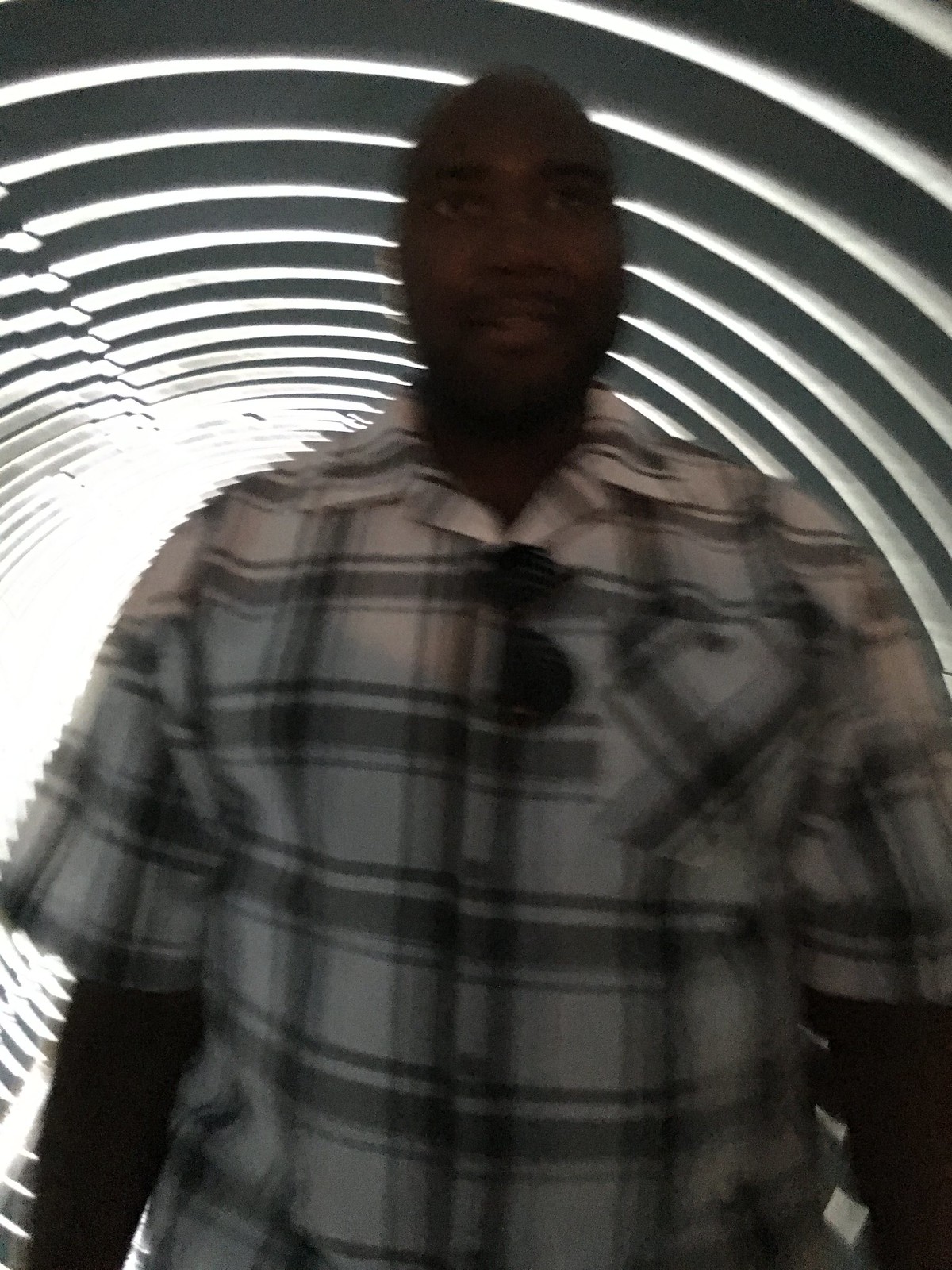In this vertically-oriented, rectangular image, we observe a grainy and blurred photograph of a man, captured from the waist up, who occupies most of the frame. The man is of African descent and is dressed in a light-colored, short-sleeve plaid shirt that is buttoned down with a collar. He is standing in what appears to be a narrow tunnel. However, there is a peculiar, jagged appearance around the edges of his shirt, suggesting he may have been digitally inserted into the scene, although the lighting in the tunnel could also explain the unusual effect. The tunnel is lit by a series of round, circular lights that are visible from the bottom to the top of the image, providing a sense of depth and perspective as the light emanates from behind the man, stretching forward into the tunnel.